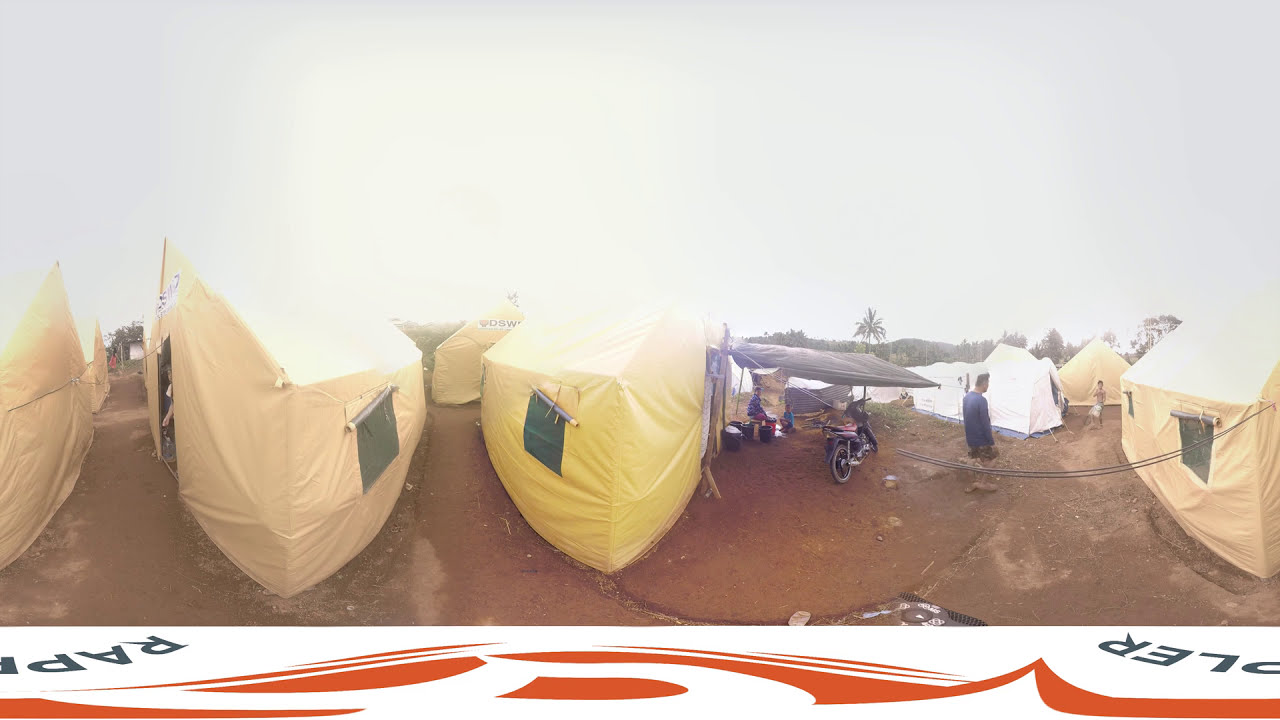The image depicts a panoramic, distorted view of a refugee camp or a camp for those displaced by a natural disaster. Spanning a horizontal frame, the scene is dominated by rows of small, light beige or light tan tents, each featuring a dark green window flap. The tents are set upon a wet, dark brown, sandy area. In the center of the image stands a distinct yellow tent, with a black awning under which sits a woman with her child beside a few buckets, possibly doing laundry. Nearby, a man in a long-sleeve bluish-gray shirt stands next to an old motorcycle. Another figure, possibly a child, is seen walking toward him. On the far right, there are several white tents completing the picture of this makeshift "tent city." Additionally, just left of the center yellow tent, one tent bears the marking "DSW" on its top.